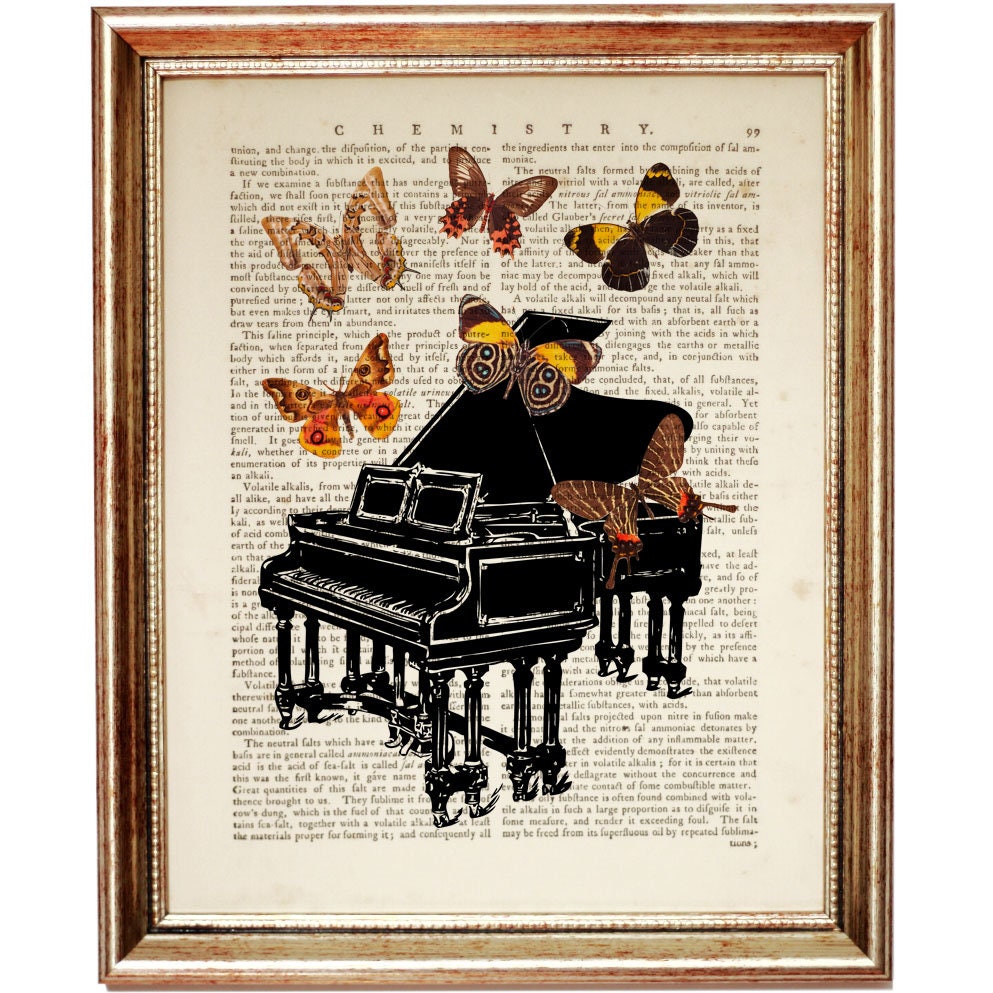This detailed and visually intricate art print is elegantly mounted in a rustic wooden frame. The background of the piece features a slightly weathered, off-white page with sepia-toned text, presumably from an old chemistry textbook, as indicated by the word "CHEMISTRY" prominently displayed at the top in classic, spaced-out black letters. The page number “99” is visible, enhancing its vintage appeal.

Prominently overlaid is a stylized black grand piano, its lid gracefully open, and the keys facing left. Adding a touch of whimsy and vibrance to the composition are six butterflies of various sizes and colors – including shades of brown, orange, black, and yellow, with intricate patterns and hints of blue. These butterflies, appearing larger than life against the scaled-down piano, float and scatter around the instrument, contributing to a surreal and imaginative scene.

The artwork embodies a harmonious blend of classical music and natural beauty, all set against an intellectually intriguing backdrop of chemical text, making it a unique decorative piece.